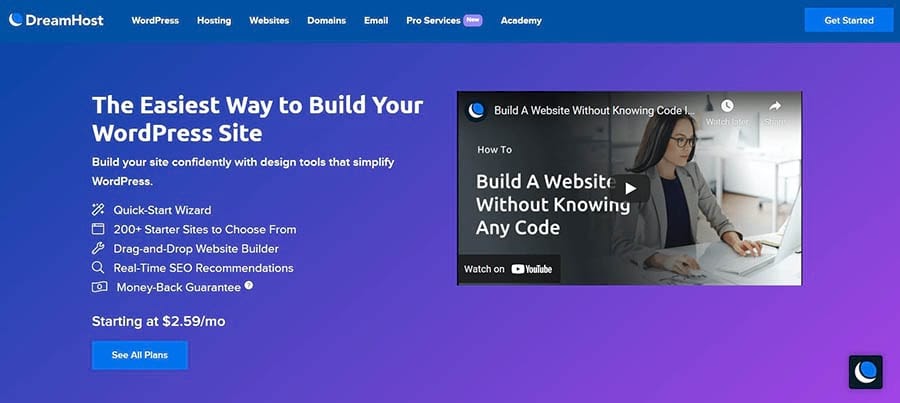This is a detailed description of a screenshot from the DreamHost website. The page features a gradient background that transitions from blue on the left to purple on the right, with a slight diagonal fade about halfway across the page. At the top, a horizontal grayish-blue banner stretches across the width of the screen, displaying the DreamHost logo and title.

The navigation menu offers several options including WordPress Hosting, Websites, Domains, Email, Pro Services, and Academy. Positioned at the upper right corner, a prominent blue button labeled "Get Started" invites users to begin their experience.

On the center-right side of the page, a video titled "Build a Website Without Knowing Code" catches the eye. The video depicts a woman with shoulder-length dark hair and light skin, wearing glasses, a gray suit jacket, and a black shirt. She is sitting at a white desk with a white laptop open in front of her, oriented to the right.

To the left, the text emphasizes the ease of building a WordPress site with DreamHost: "The Easiest Way to Build Your WordPress Site. Build your site confidently with design tools that simplify WordPress." Key features are highlighted, including a Quick Start Wizard, over 200 starter sites to choose from, a drag-and-drop website builder, and real-time SEO recommendations. A money-back guarantee is mentioned, with pricing starting at $2.59 per month. Below this, a blue button labeled "See All Plans" provides further options for interested users.